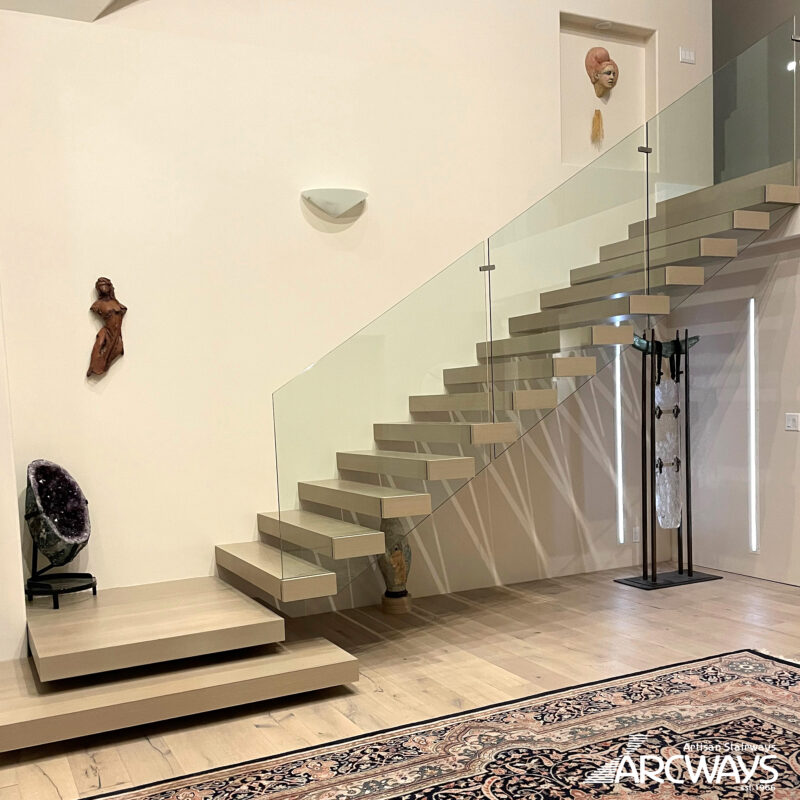This is a detailed interior photograph of a stairwell inside a commercial building, watermarked ARCWAYS in the bottom right corner. The staircase appears to be floating, with individually mounted steps that look like they are made of smooth, reflective metal, perhaps giving a floating illusion emanating from the wall. The steps are complemented by a sleek glass railing. On the floor, there is an ornate Persian rug.

At the base of the stairs, in the corner, stands a large, split purple geode, emanating a striking presence. Ascending the staircase, various pieces of art are prominently displayed. Notably, there is a brown, rust-colored statue of a woman’s torso without arms or legs, mounted seamlessly onto the wall. A wall sconce provides illumination nearby. Higher up, embedded within a rectangular depression in the wall, sits another sculptural piece: a head of a woman, detailed with hair intricately styled atop her head. The walls, pristine in white, create a perfect backdrop for this eclectic artistic display, enhancing the overall aesthetic of the pristine, contemporary space.